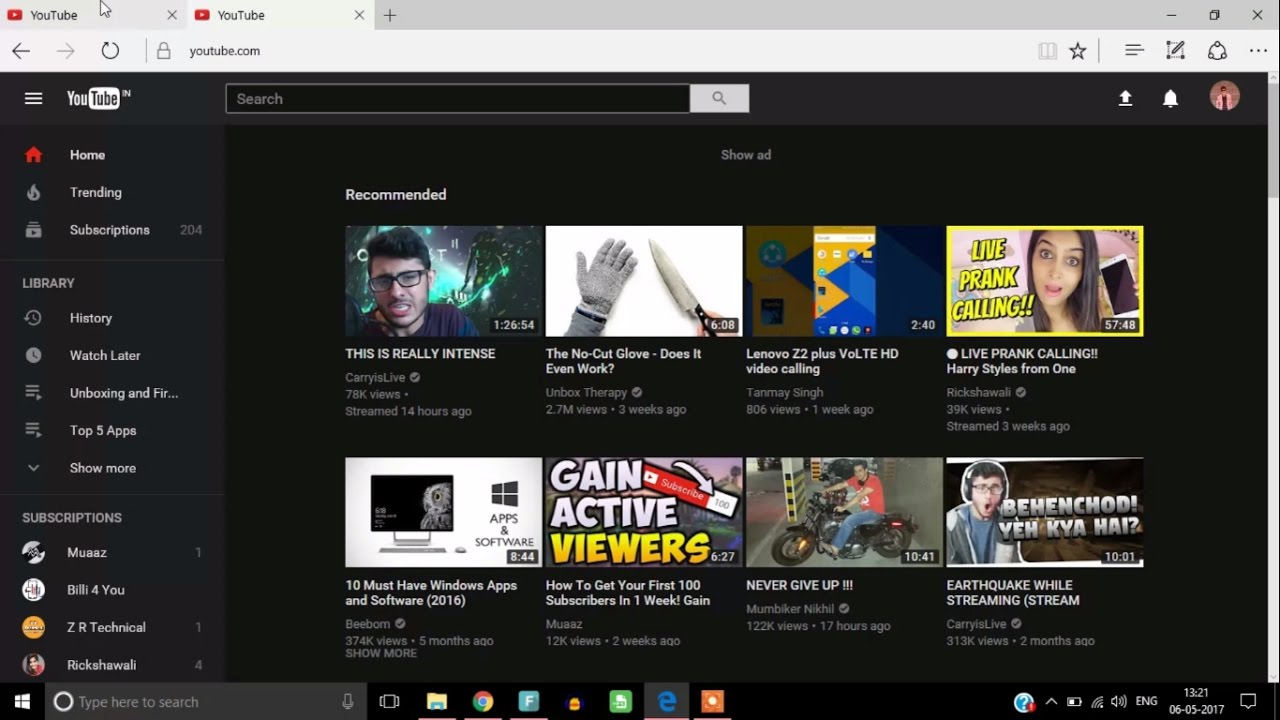The image is a screenshot of a Windows operating system desktop displaying an open Internet Explorer browser window. 

The Internet Explorer window showcases two tabs, both labeled "YouTube." The URL in the address bar is YouTube.com, and the interface includes standard navigation elements: a back button, a refresh icon, and an X button to close the window. The browser window is set against a predominantly gray background.

At the bottom left of the screen, the Windows taskbar displays the familiar Windows logo next to a search bar labeled "Type here to search." To the right of the search bar are several application shortcuts, including a yellow folder icon (possibly for File Explorer), the Google Chrome icon, an "F" (potentially for Facebook), and another unknown icon. An "E" icon suggests that Internet Explorer is the active browser. Further right on the taskbar, there are system icons for battery status (without a percentage), Wi-Fi signal strength, volume control, and a language setting labeled "ENG."

The system clock shows the time as 13:21, with the date marked as 06/05/2017.

The centerpiece of the browser window is the YouTube homepage, featuring recommended videos against a predominantly black background. Visible video titles include: "This is really intense, Vicarious Live" with 78,000 views, streamed 14 hours ago; "The No-Cut Glove, Does it Even Work?"; and "Lenovo Z2 Plus, VoLTE HD Video Calling." Additionally, there is a video on the right side titled "Live Prank Calling Harry Styles from One."